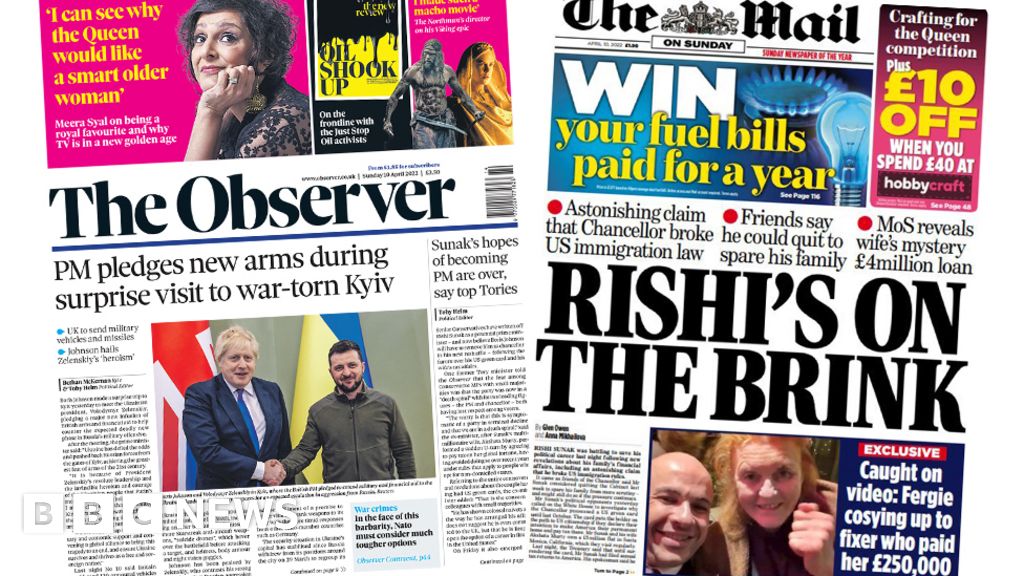Displayed side-by-side are the front pages of two British newspapers. On the left is the Daily Mail, and on the right is The Observer, both dated April 10th, 2023, though the exact date is slightly blurry. 

The main headline of The Observer features, "PM Pledges New Arms During Surprise Visit to War Torn Kiev," accompanied by a photograph of Boris Johnson shaking hands with President Zelensky. 

The Daily Mail's primary headline screams, "Rishi's on the Brink," with three sub-headlines marked by red spherical icons: 
- On the left: "Astonishing Claim that Chancellor Broke U.S. Immigration Law."
- In the middle: "Friends Say He Could Quit to Spare His Family."
- On the right: "MOS Reveals Wife's Mystery £4 Million Loan."

Both newspapers feature various other articles and colorful advertisements. The Observer and the Mail provide a stark contrast in their focal stories, one highlighting international diplomacy and the other embroiled in domestic political scandal.